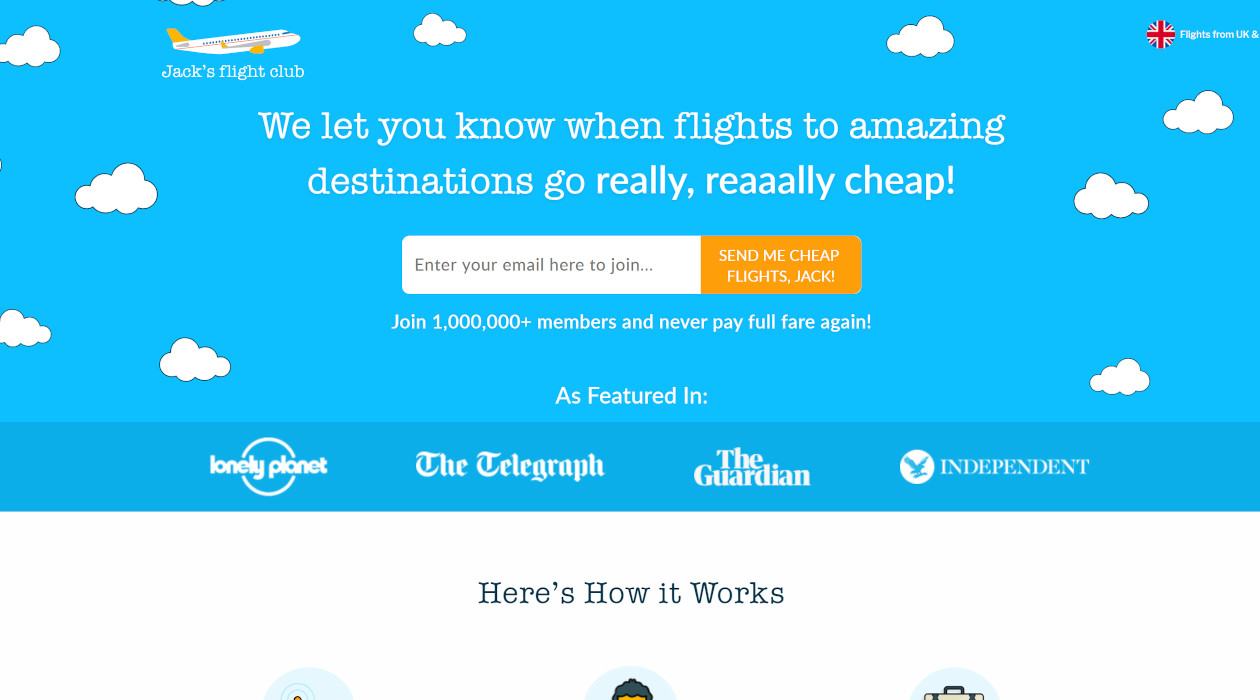This screenshot showcases the vibrant homepage of Jack's Flight Club, predominantly featuring a blue background adorned with cartoonish white, fluffy clouds, creating a whimsical flight theme. Dominating the upper section, a playful airplane soars above the bold white text "Jack's Flight Club." Adjacent to this, partial text reads "Flights from UK an..." with the remaining words cut off.

Centrally positioned in large, white, and playful text is the club's enticing promise: "We let you know when flights to amazing destinations go really, really cheap," with the second "really" humorously elongated as "R-E-A-A-A-L-L-Y." Below this, a prominent email sign-up area invites users to join, highlighted by the placeholder text "Enter your email here to join" within a white input box. Adjacent to this, a striking gold button urges visitors with the call to action: "Send me cheap flights, Jack."

Further down, the text "Join one million plus members and never pay full fare again!" enthusiastically encourages membership. Beneath this, the section labeled "As featured in" is followed by an array of reputable logos: Lonely Planet, The Telegraph, The Guardian, and The Independent, all neatly aligned on a slightly darker blue bar.

The final segment visible in the screenshot starts with the text "How it works," suggesting further insights into the club’s operational details lie below.